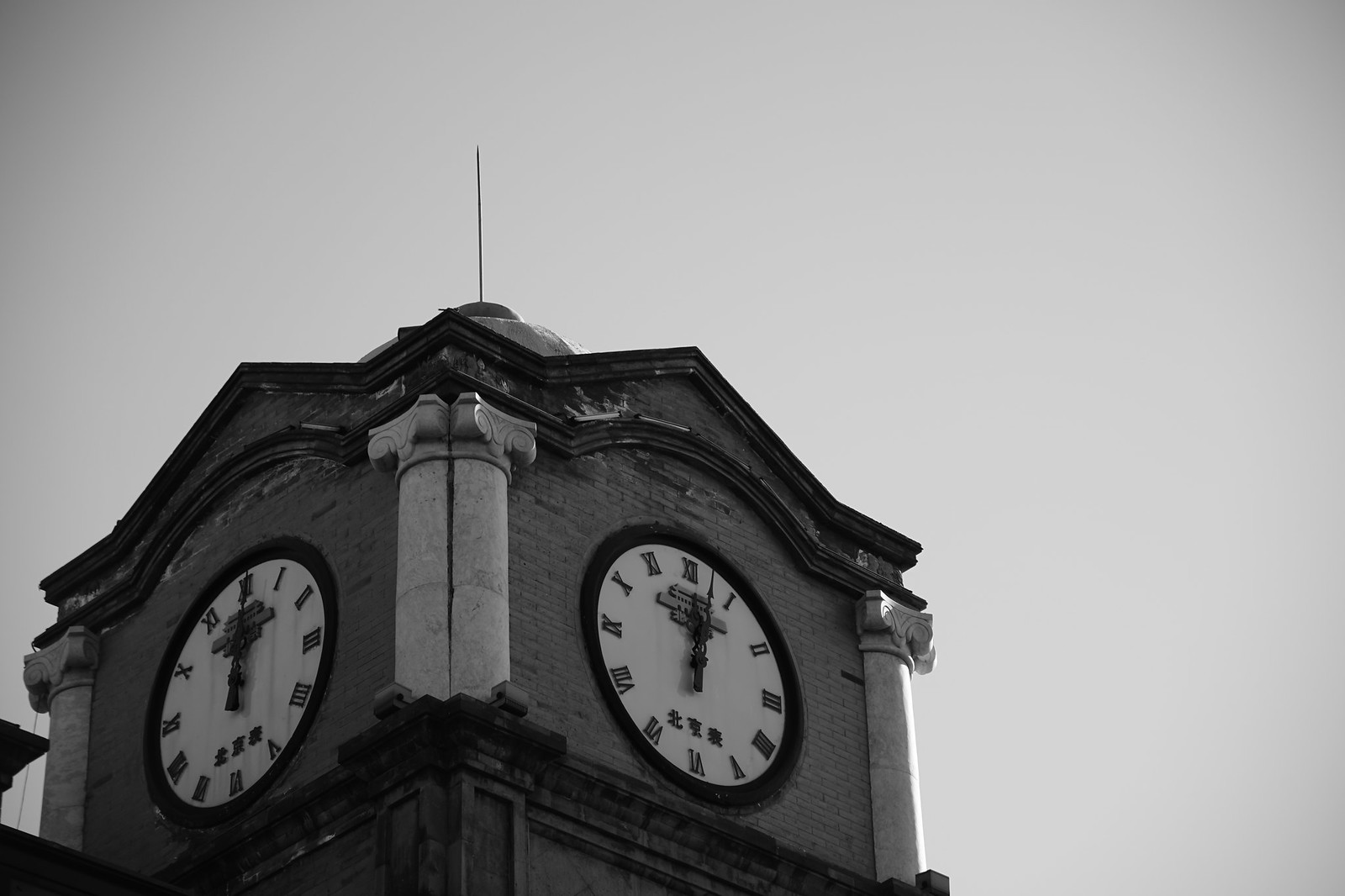This black and white photograph captures a towering clock tower, viewed from ground level with the sky as a backdrop. The structure features four sides, with prominently visible clocks on two of them, each adorned with Roman numerals and both indicating the time as noon. The architectural style of the tower suggests a blend of Victorian and Renaissance influences, evoking a sense of historical grandeur. An antenna perches atop the tower, adding a touch of modernity to the old-world charm. The sky above appears relatively clear, though there is a subtle, possibly gloomy undertone to the atmosphere.